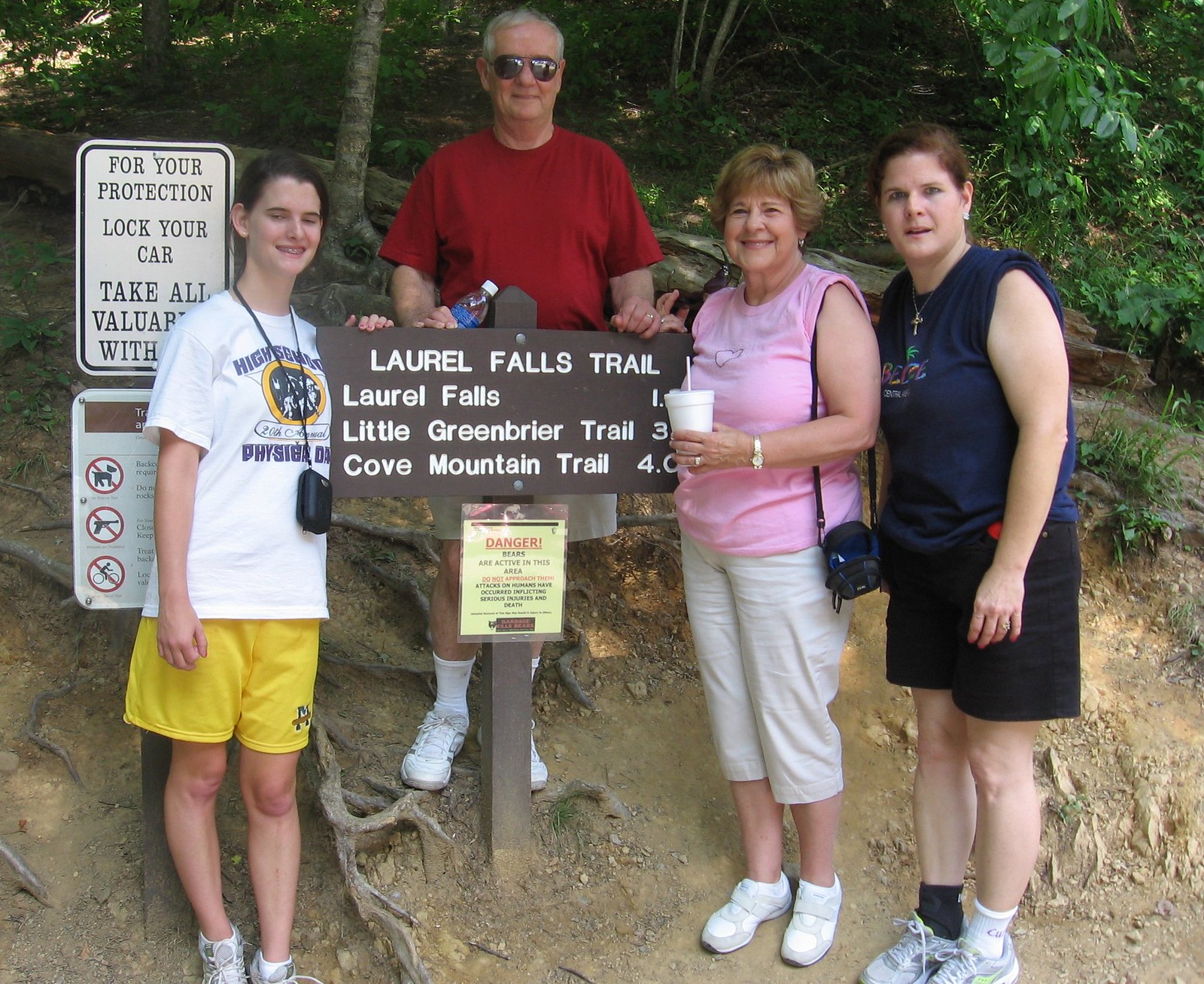In this outdoor image, likely taken in a park, four people stand around a prominent wooden sign that marks the start of the Laurel Falls Trail. The brown, wooden sign, firmly anchored in the ground, displays information in white lettering: "Laurel Falls Trail," then "Laurel Falls 1," below it "Little Greenbrier Trail," and further down "Cove Mountain Trail 4.0." A rectangular laminated sign at the bottom, in red lettering, reads "Danger."

From left to right, the individuals around the sign include a young girl wearing a white t-shirt with unreadable symbols and yellow shorts. She has white shoes on and a strap around her neck, possibly a purse or camera. To her left, the central figure, a man with gray hair and sunglasses, sports a red shirt, light brown shorts, and white sneakers. He is holding a water bottle in his right hand and has his left hand resting on the sign.

On the right side of the sign, a woman in a pink blouse with sleeves rolled up to create a tank top look, wears white capri pants and white sneakers. She holds a cup with a straw in her left hand. Behind her stands another younger woman dressed in a black dress, contrasting socks—one black and one white—and white sneakers. The background features a mix of tree trunks and foliage from bushes, adding to the natural setting. The ground at their feet is primarily dirt, indicating a well-trodden trail. Additionally, there is a metal sign nearby that reads, "For Your Protection, Lock Your Car, Take All Valuables With You."